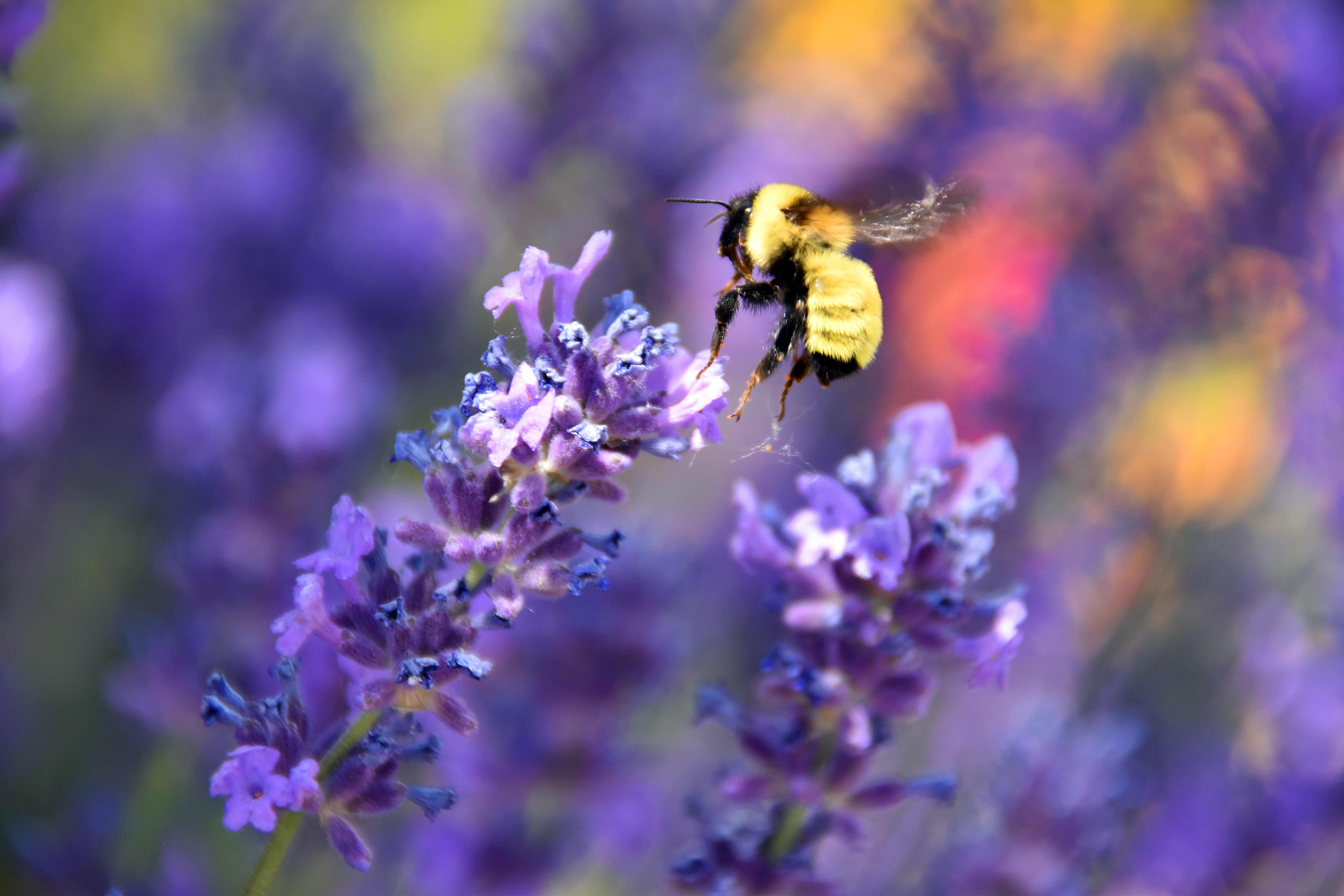This professionally taken, highly detailed close-up captures a beautiful bumblebee hovering just above two tall, narrow, purple flowering plants. The bee, characterized by its thick, yellow-backed body with distinctive black legs and black head, has a yellow patch on its neck resembling a cape. Its wings are a blur, flapping rapidly to keep it suspended in the air. The long purple flowers, resembling hot dogs on sticks, are adorned with tiny buds and florets. The image has a horizontally oriented frame, with the foreground in sharp focus and the background beautifully blurred, accentuating the bee and the flowers. The blurred backdrop is filled with hues of yellow, pinkish-orange, and more purple flowers, ensuring all attention is drawn to this meticulous interaction between the bumblebee and the purple blooms.